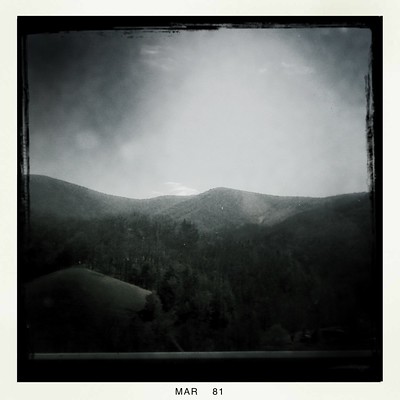The black and white photograph, dating back to March 1981 as indicated by the "MAR 81" inscription at the bottom, is bordered by a distinctly narrow black frame with an outer white border. The image captures a tranquil, early morning outdoor scene. In the foreground, there is a dense clustering of dark trees, their branches barely visible due to the faint pre-dawn light. Rising behind this arboreal expanse is a line of hills extending towards high, snow-capped mountain ranges that stretch across the horizon. The sky, predominantly white with some darker clouds on the outer edges, suggests the sun is about to rise, casting a soft glow over the terrain. Interestingly, there appears to be an object resembling a broken missile nestled amongst the trees, adding an enigmatic touch to the serene landscape.